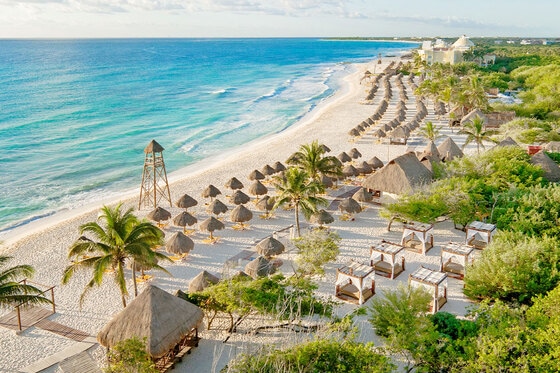This detailed image captures the idyllic scene of a tropical beach, possibly Paraiso del Mar in Mexico, taken from an elevated perspective, perhaps from a drone. In the top left corner, the aquamarine blue ocean meets the edge of the white sandy shore, which runs diagonally from center left to top right. The sandy beach is bustling with numerous straw-topped triangular huts, open on all sides, and multiple rows of beach chairs and rattan umbrellas, likely rentals, creating a busy yet orderly scene. Dominating the right-hand side are the palm trees that dot the shore, with their density increasing as the eye moves inland. In the background, a cluster of lush green trees forms a dense canopy, creating a natural boundary. Here, several canopy beds, resembling four-poster beach huts, are nestled among the trees, adding to the tropical ambiance. Toward the top right, just beneath the horizon, a large white building with domed structures is visible, standing majestically in the distance. This picturesque beach, with its arranged umbrellas, cabanas, and tiki hut structures, reflects a serene yet vibrant tourist destination, exuding an exotic charm reminiscent of South Pacific islands, albeit without a single person in sight.